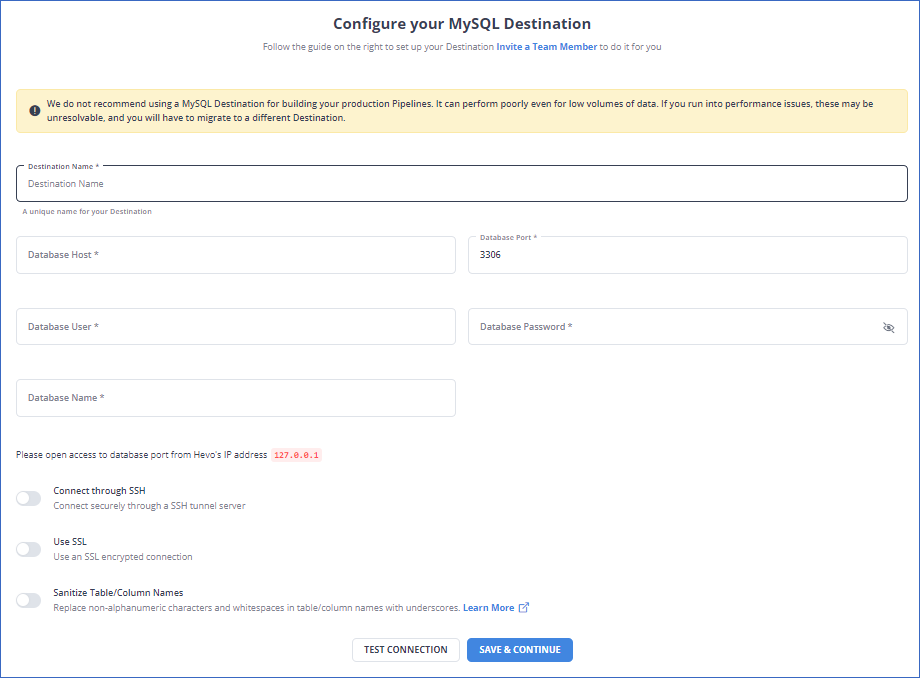This image showcases the configuration interface for setting up a MySQL destination on a website or application. The interface is visually framed with a thin blue border and predominantly consists of input fields and instructions. At the top, there is an important note advising users to follow the period to the right of the destination, especially when delegating the task to a team member.

Beneath this note is a highlighted disclaimer in a yellowish-tan box, cautioning against the use of MySQL destinations for production pipelines due to potential performance issues. It advises users that volume handling could be problematic and migrating to an alternative destination might be necessary if performance issues arise.

Below the disclaimer are various fields to configure the MySQL destination. The first field is a long text box for naming the setup. Following this are multiple input boxes for essential connection details: the host, user name, database name, port number (pre-filled with "30306"), and password. Additionally, there is an option to open access to the database port, along with the option to enter an IP address and toggle various settings. These settings include connecting via SSH, using SSL for connection security, and specifying table column names.

At the bottom center of the box, users are provided with two actionable buttons: "Test Connection" to verify the setup or "Save and Continue" to proceed with the configuration.